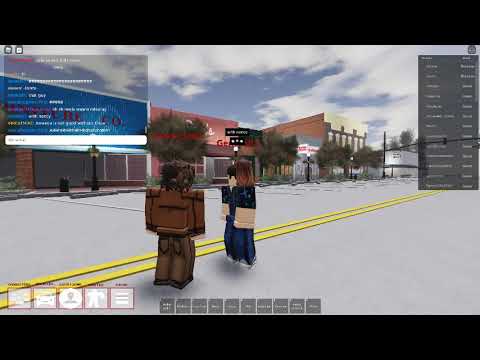The image is a screenshot from the game Roblox, featuring a vibrant digital world. It has black bars at the top and bottom, framing the scene. The terrain is a gray road with a yellow dashed line running diagonally from the bottom left to the upper right. Centered on the road are two blocky, LEGO-like characters: one on the left with brown hair, dressed entirely in brown, and the other to the right in a blue jumpsuit with peach-colored skin and brown hair. 

Behind them, a row of colorful shop buildings and trees stretches across the top two-thirds of the image. The buildings exhibit a range of colors, including salmon, brown, tan, and gray, while the sky above is a vivid blue dotted with white clouds. There's a faint, unreadable group chat situated in a gray box at the top left corner, and the bottom center of the screen features several gray buttons. The overall composition suggests a scene within a bustling virtual street, highlighting the game's stylized, 3D block-like aesthetic.